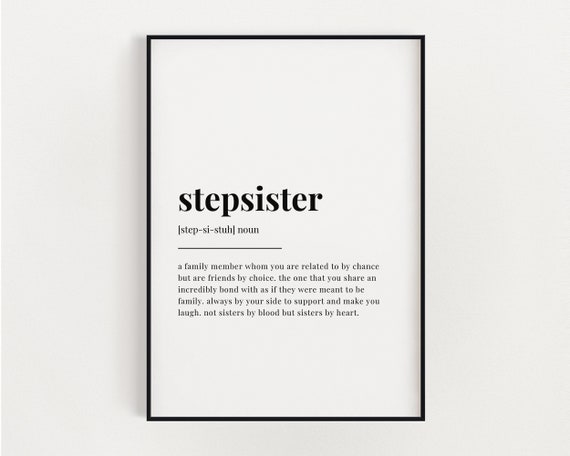The image depicts a black-framed poster on completely white paper, resembling a definition entry. The large header "stepsister," all in lowercase letters, is bold and centered at the top. Below it, in brackets, is the pronunciation guide: [step-sis-ter]. The entry labels the term as a noun, followed by a horizontal line stretching from the first 's' in "stepsister" to the second 't'. Beneath the line, the definition reads: "a family member whom you are related to by chance, but are friends by choice. The one that you share an incredible bond with, as if they were meant to be family. Always by your side to support and make you laugh. Not sisters by blood, but sisters by heart." Each sentence begins in lowercase letters, emphasizing an intimate, informal tone.